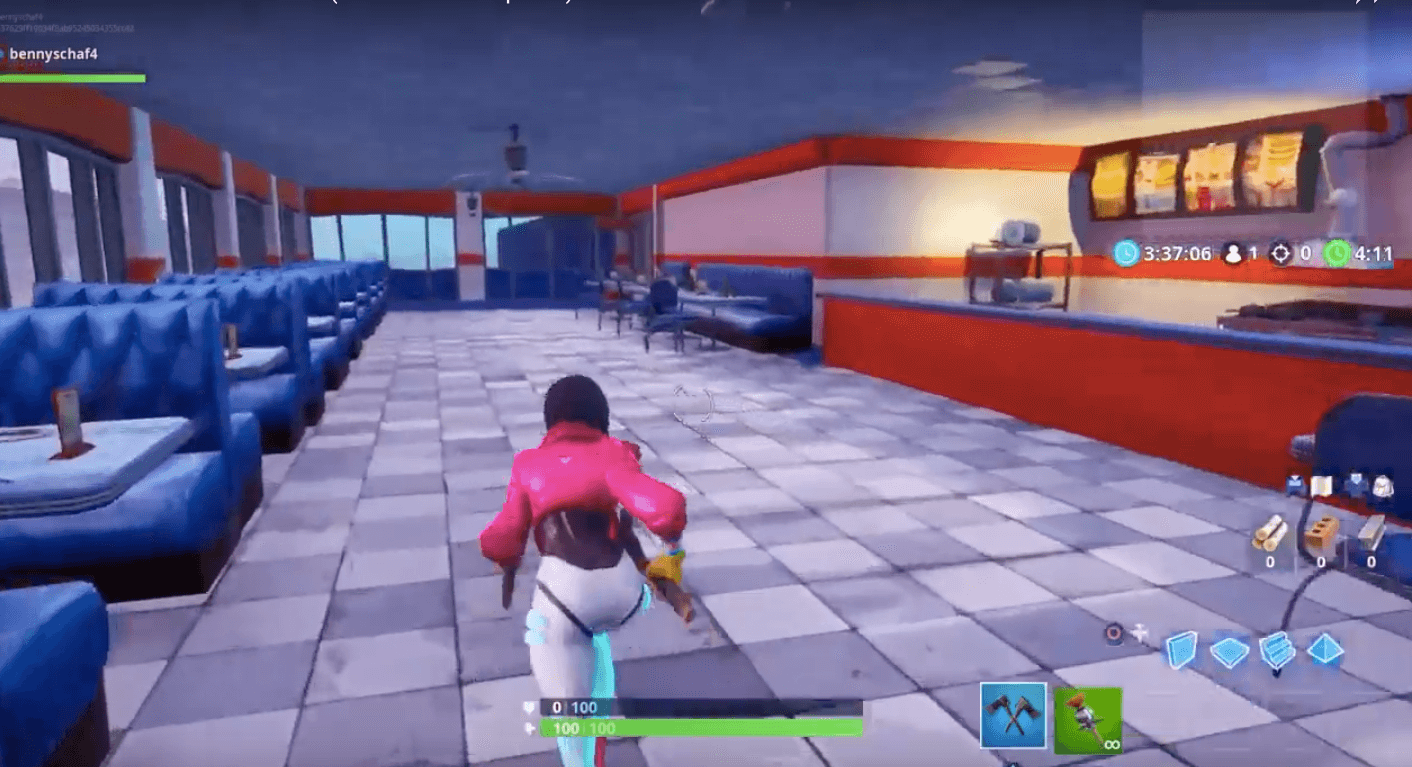The image is a screen grab from a video game, depicting the interior of a fast-food restaurant. Dominating the left side is a row of blue padded booths extending from the bottom left corner to the distant end of the establishment, with windows visible between some of the booths. The ceiling has a grayish hue and the floor showcases a light gray and dark gray alternating tile pattern. Central to the image is an animated character with black hair, possibly styled in a bob or covered by a black helmet. Wearing a pink puffy jacket, white skin-tight pants, and yellow gloves, the character is seen moving away from the viewer, with an axe in one hand and possibly another object in the other. Their skin appears to be brown. At the bottom of the image, across the character's legs, are two status bars—one gray and one green—marked with numbers, likely representing health or status indicators. To the right, we see an orange counter with a blue top, accompanied by what seems to be an illuminated yellow menu. Above the counter are various icons and numbers, suggesting interactive elements or options in the game.